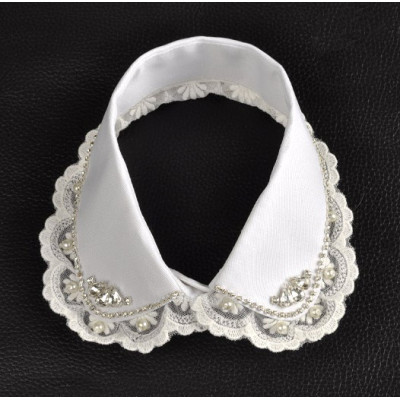This image presents an isolated, ornate white collar set against a stark black background, possibly leather. Central in the composition, the collar appears pristine and is distinguished by its intricate frilly pattern along the edges, transitioning into a smooth white interior. The elaborate embellishments include diamond-shaped designs, spiral motifs, floral patterns, and possibly small crystals or pearls adorning the sides. The strong contrast between the black background and the pure white collar heightens its visual appeal, suggesting it is a luxurious and historic item, likely from over a century ago, indicative of high social status. The image evokes the setting of a museum display, accentuated by the simplicity and elegance of the scene. There is no text present in the image, emphasizing the collar's artistic and historical significance.